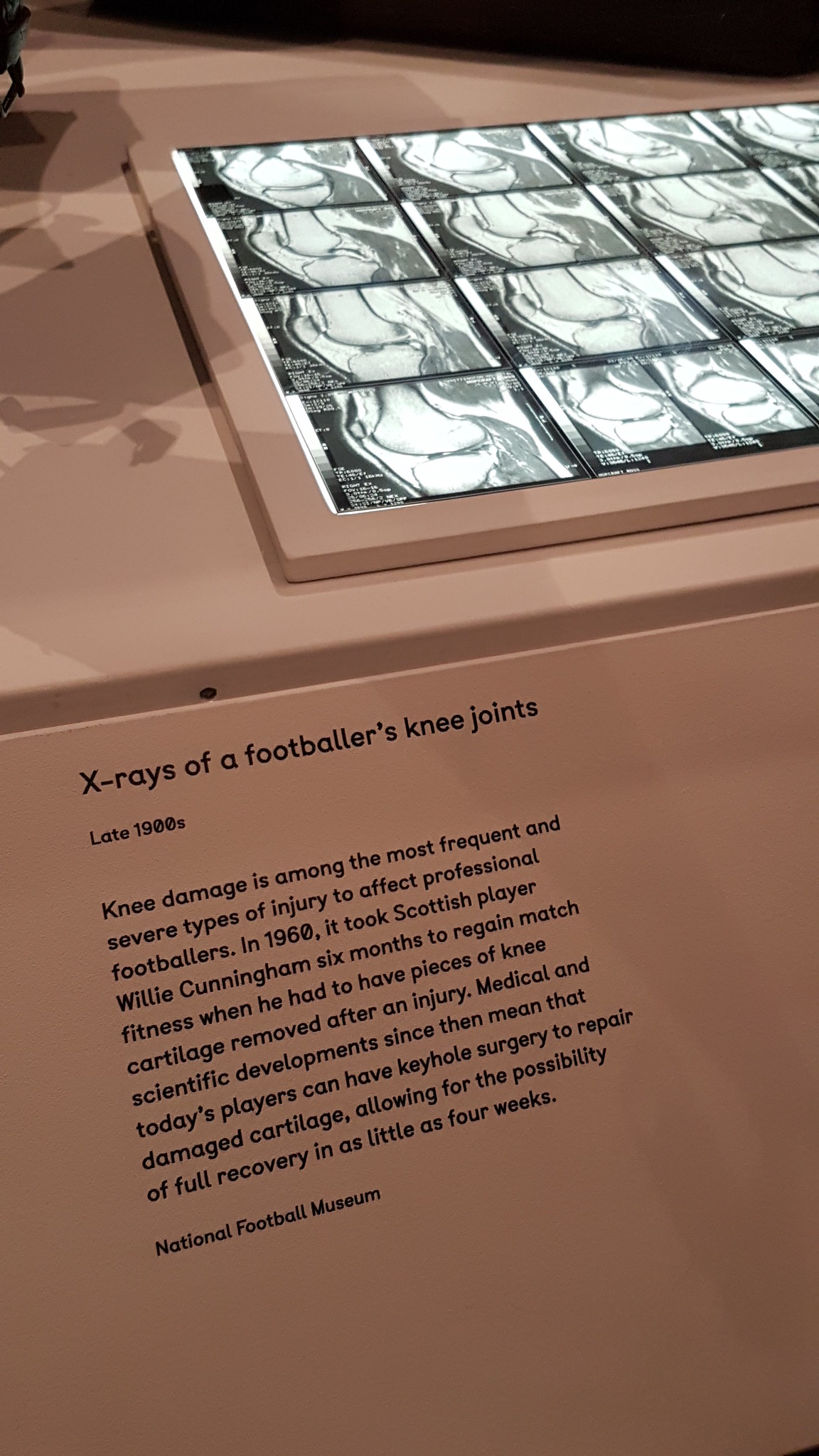The image depicts a museum display at the National Football Museum, featuring a wooden table with integrated x-ray images and informational text about football-related knee injuries. The top section of the display, mounted on a sloping downward panel, showcases at least 16 x-ray images of knee joints, likely from the late 1900s. Below these images, the text explains that knee damage is among the most severe injuries suffered by professional footballers. It highlights the case of Scottish player Willie Cunningham, who took six months to recover match fitness after knee cartilage removal in 1960. Advances in medical and scientific techniques since then have enabled today's players to undergo keyhole surgery, potentially achieving full recovery within four weeks. The display emphasizes the evolution of treatment methods for knee injuries in football.